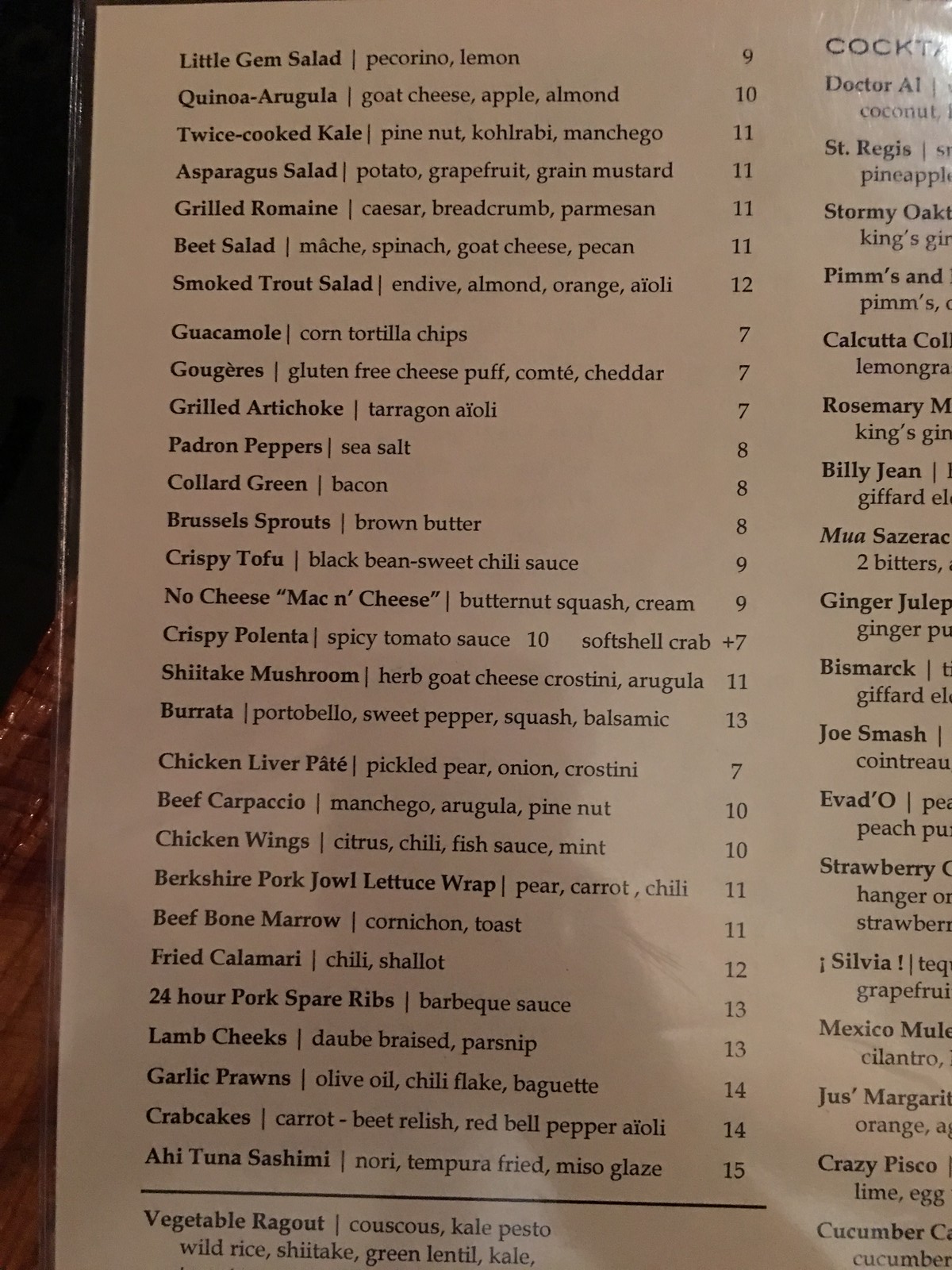The image depicts a section of a restaurant menu, featuring a clean, white background with black text, all laminated. The lamination is slightly peeling from the left side of the menu. At the top of the menu are various salad options listed as follows:

- Little Gem Salad with Peppercorn and Lemon - $9
- Quenado Arguinas with Goat Cheese, Apple, and Almond - $10
- Twice Cooked Kale with Pine Nut and Manchego - $11
- Asparagus Salad with Potato, Grapefruit, and Grain Mustard - $11
- Grilled Romaine Caesar with Bread Crumb and Parmesan - $11
- Beet Salad with Ismache, Spinach, Goat Cheese, and Pecan - $11
- Smoked Trout Salad with Endive, Almond, Orange, and Aloe - $12

There are additional items such as Guacamole with Corn Tortilla Chips, and a dish with a Spanish word “Gougeres.” The menu continues with various appetizers and dishes like:

- Grilled Artichoke
- Pedron Peppers
- Brussel Sprouts
- Crispy Tofu
- No Cheese Mac and Cheese
- Crispy Polenta
- Shiitake Mushroom
- Burrata
- Chicken Liver Pâté
- Beef Carpaccio
- Chicken Wings
- Bouchard Pork Jowl
- Beef Bone Marrow
- Fried Calamari
- 24 Hour Pork Spare Ribs
- Lamb Cheeks
- Garlic Ponds
- Crab Cakes
- Ahi Tuna Sashimi

The detailed list indicates a diverse offering of salads, small plates, and main dishes designed to cater to a variety of tastes and dietary preferences.